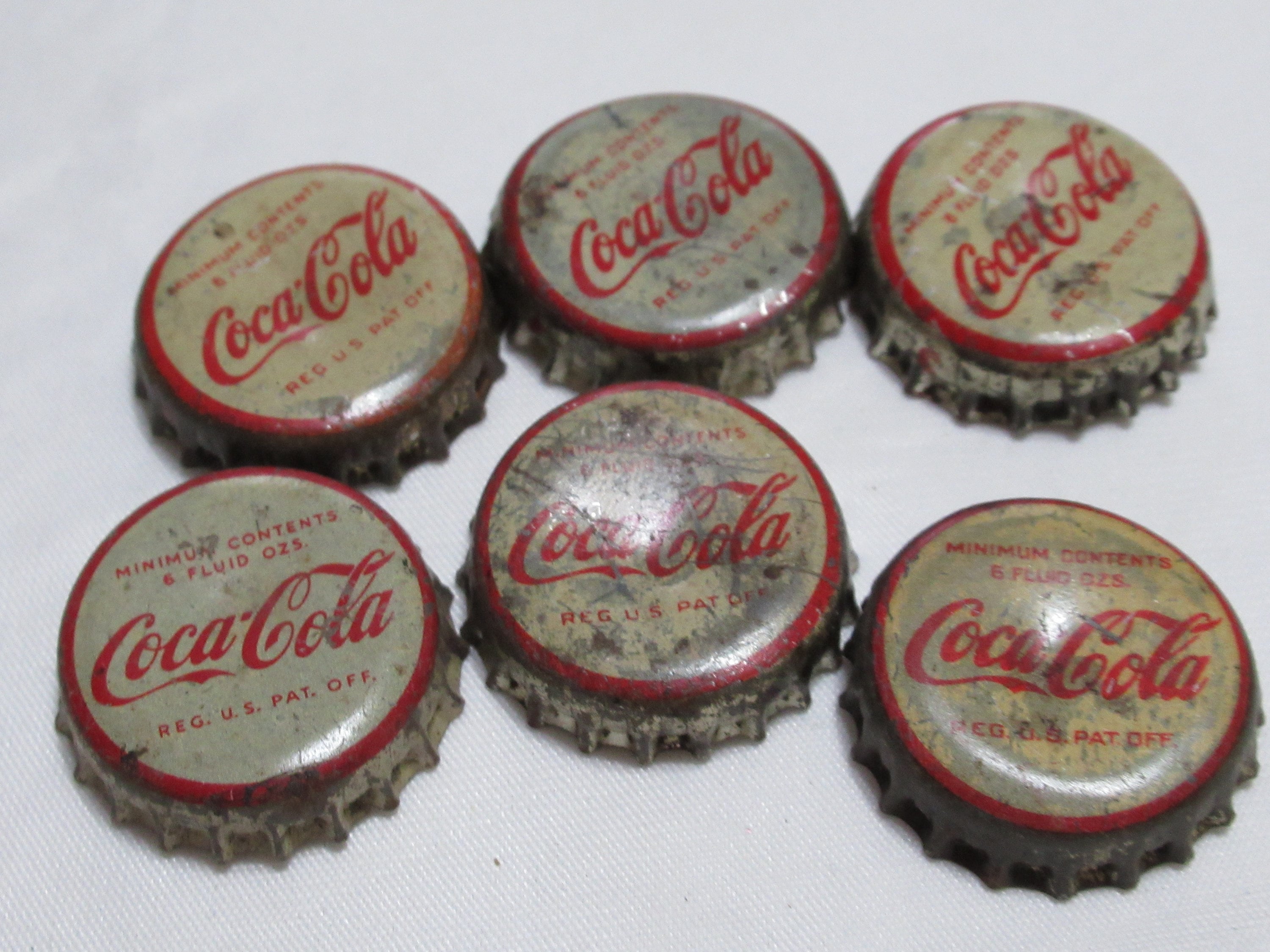This is a detailed picture of six old and weathered Coca-Cola bottle caps. Arranged symmetrically on a white textured tablecloth, the bottle caps form two rows of three each, all facing upward with the ridged sides down. Once white, these metal caps now appear a faded light gray or cream due to extensive wear and tear. The design includes a red ring bordering the cap's circumference. In red font at the top, they display the wording "Minimum Contents Six Fluid OZS," followed by the iconic Coca-Cola scripted logo. Beneath the logo, also in red, is the text "Reg. U.S. Pat. Off." The caps exhibit varying degrees of paint loss and scratches, with the two on the left being in relatively better condition than the rest.